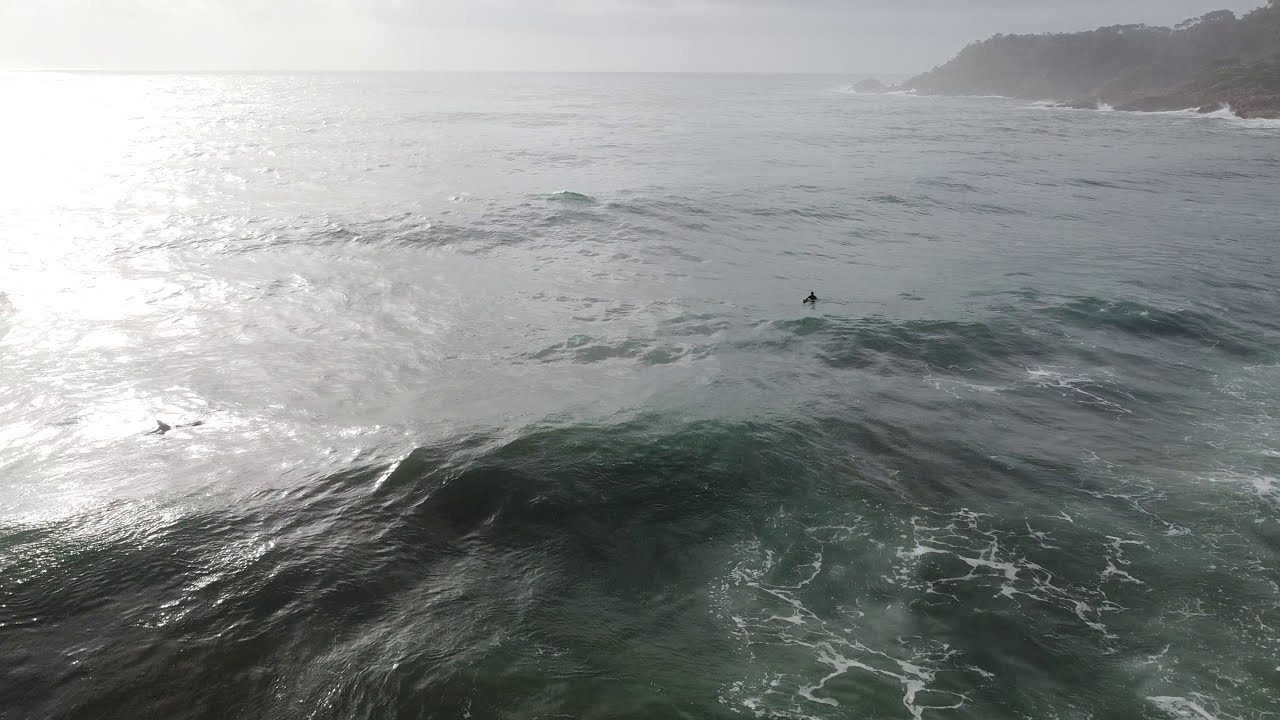This top-down photograph captures a serene ocean scene, featuring two distant surfers donned in what appears to be all black. One surfer is positioned towards the left side of the image, while the other is located around the right middle portion, with the tip of his surfboard slightly visible above the water's surface. The ocean itself presents mild waves, better described as gentle swells or "water speed bumps," with patches of white foam evident, particularly near the bottom right of the image close to the coastline. The water transitions from a deep turquoise to almost black in some areas, gradually lightening towards the horizon where the overcast sky takes on a pale gray hue. In the top right, a mountainous landscape adorned with trees emerges from the fog, sloping down towards the water. The left side of the image is subtly lit by sunlight filtering through, casting a gentle glare across the scene, enhancing the tranquil yet slightly stormy atmosphere.